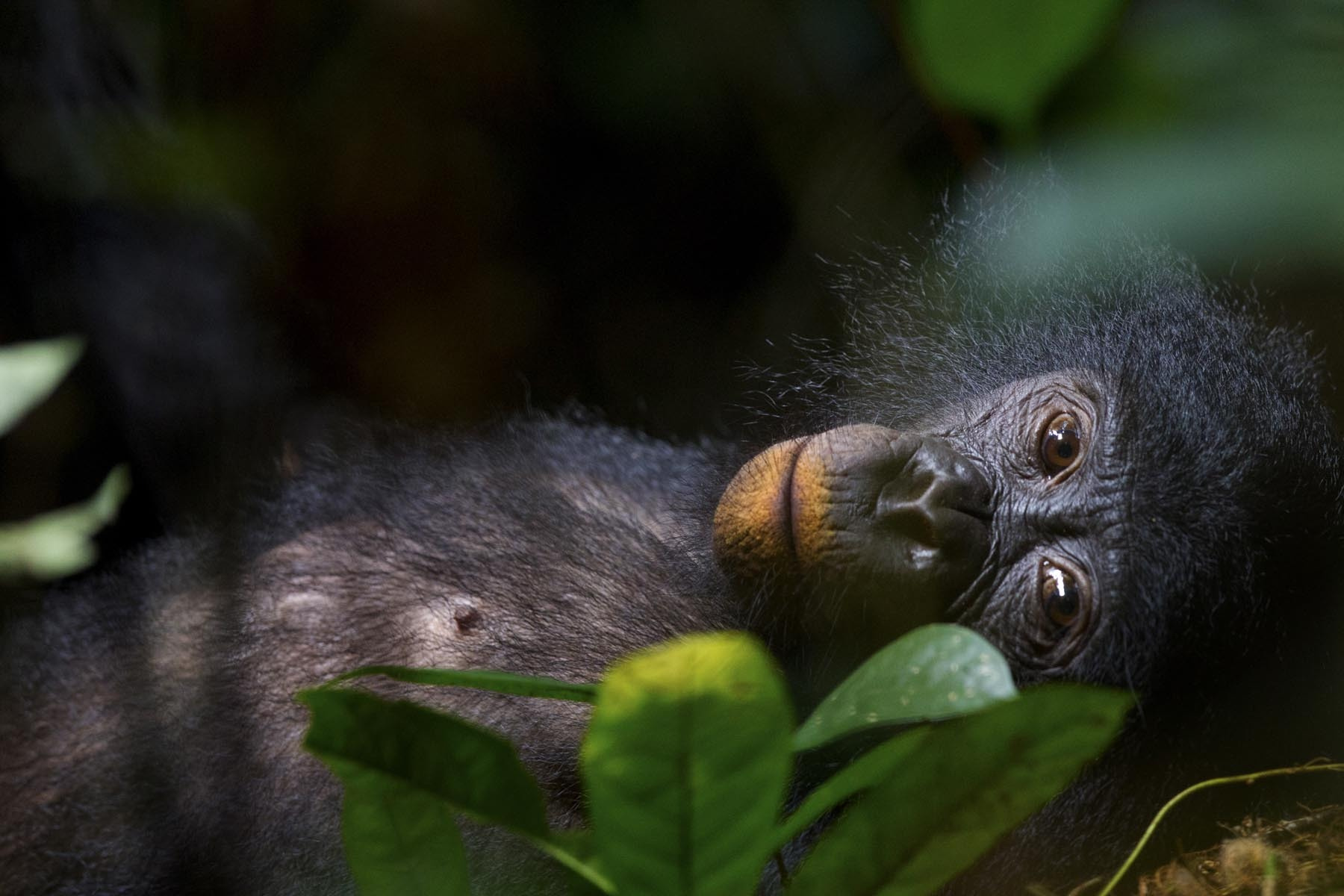In this image, a primate, specifically a monkey, is depicted lying down in a natural forest setting. The scene focuses primarily on the monkey's face and chest as it looks directly at the camera, embodying a calm, relaxed state with a touch of melancholy. The monkey has striking brown eyes, a black nose, and distinct black fur with some exposed flesh on its chest. Its mouth area is brown with a golden-yellow tint that resembles makeup. The background is predominantly black with blurred green foliage on the upper right-hand side and at the bottom, where bright green plants stand out more clearly. A few twigs and vines are also visible, contributing to the jungle-like ambiance. The lighting focuses on the monkey, suggesting it might be nighttime, yet the illumination casts a gentle glow on its fur. The head positioned to the right and the chest to the left, along with the blurred backdrop, accentuate the primate as the central element of the photograph.